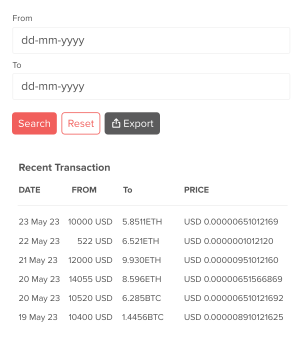The webpage features a minimalist design set against a white background. At the very top left corner, there is a section for specifying a date range, labeled "From" and "To." Each label is accompanied by a text input box allowing dates to be entered in the format "dd-mm-yyyy".

Below the date range section, there are three buttons aligned horizontally from left to right. The first button is red with the word "Search" prominently displayed in white text. The second button is white with a red border and features the word "Reset" in red. The third button is black, displaying the word "Export" in white along with a white download icon.

Directly underneath these buttons, the section header "Recent Transactions" is displayed in bold black text. This section is organized into four vertical columns labeled "Date," "From," "To," and "Price." Beneath these headers, there are six rows of data detailing recent transactions, each row corresponding to these categories.